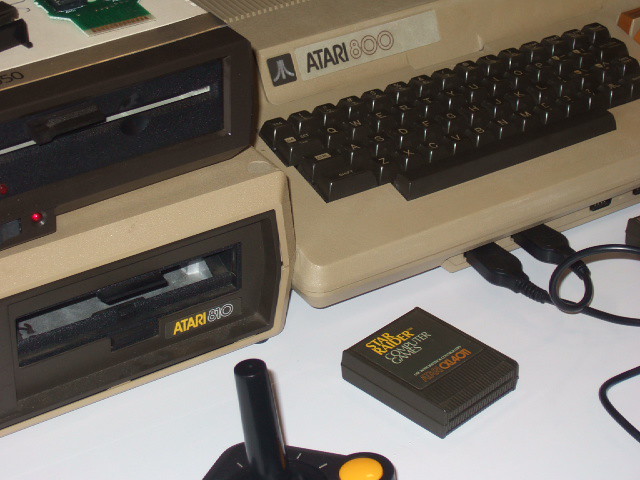The image showcases vintage Atari computer hardware, slightly wider than it is tall, approximately by 30%. Dominating the right side is the Atari 800, identifiable by a clearly visible Atari logo and label above the left-hand side of its black keyboard. This computer-console hybrid, dating back to the late 70s or early 80s, shows two black cords, likely from controllers, plugged into the front of the keyboard, though the controllers themselves are not shown.

To the left, there is an Atari 810 disk drive, a light brown unit about three inches tall with a notable black area for disk insertion. Above this disk drive is another similar unit with a red button on it. Positioned toward the center is a game cartridge, angling toward the upper left corner, labeled "Star Raider." Nearby, a classic Atari joystick with a single button rests, adding to the nostalgic ambiance of the vintage gaming setup.